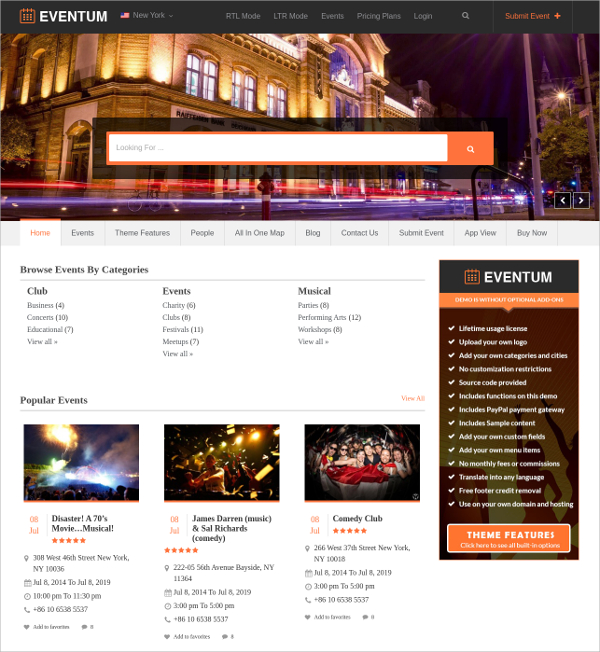The webpage titled "Eventum" serves as a comprehensive calendar platform, allowing users to both discover and organize local events. The site features a sleek black bar with white lettering across the top, providing various options such as "New York," "RTL mode," "LTR mode," "Events," "Pricing," "Plans," "Login," "Search," and "Submit Event." 

A striking panoramic image of a lit-up building is prominently displayed, encapsulated in a white box with orange borders. Below this, menu buttons offer quick navigation to "Home," "Events," "Theme Features," "People All on One Map," "Blog," "Contact Us," and submission and viewing options for events.

Users can browse events by categories like charity, clubs, parties, and performing arts among others. The section for popular events features highlights such as "Disaster, a 70s Movie American Musical," "James Darren Music," "Sal Richards Comedy," and a "Company Club" option. 

On the right side, there's a buy-in section showcasing nearby events and thematic features, aiding users in organizing or discovering local activities. Eventum appears to be a versatile calendar assistant designed for both event setup and local event discovery.